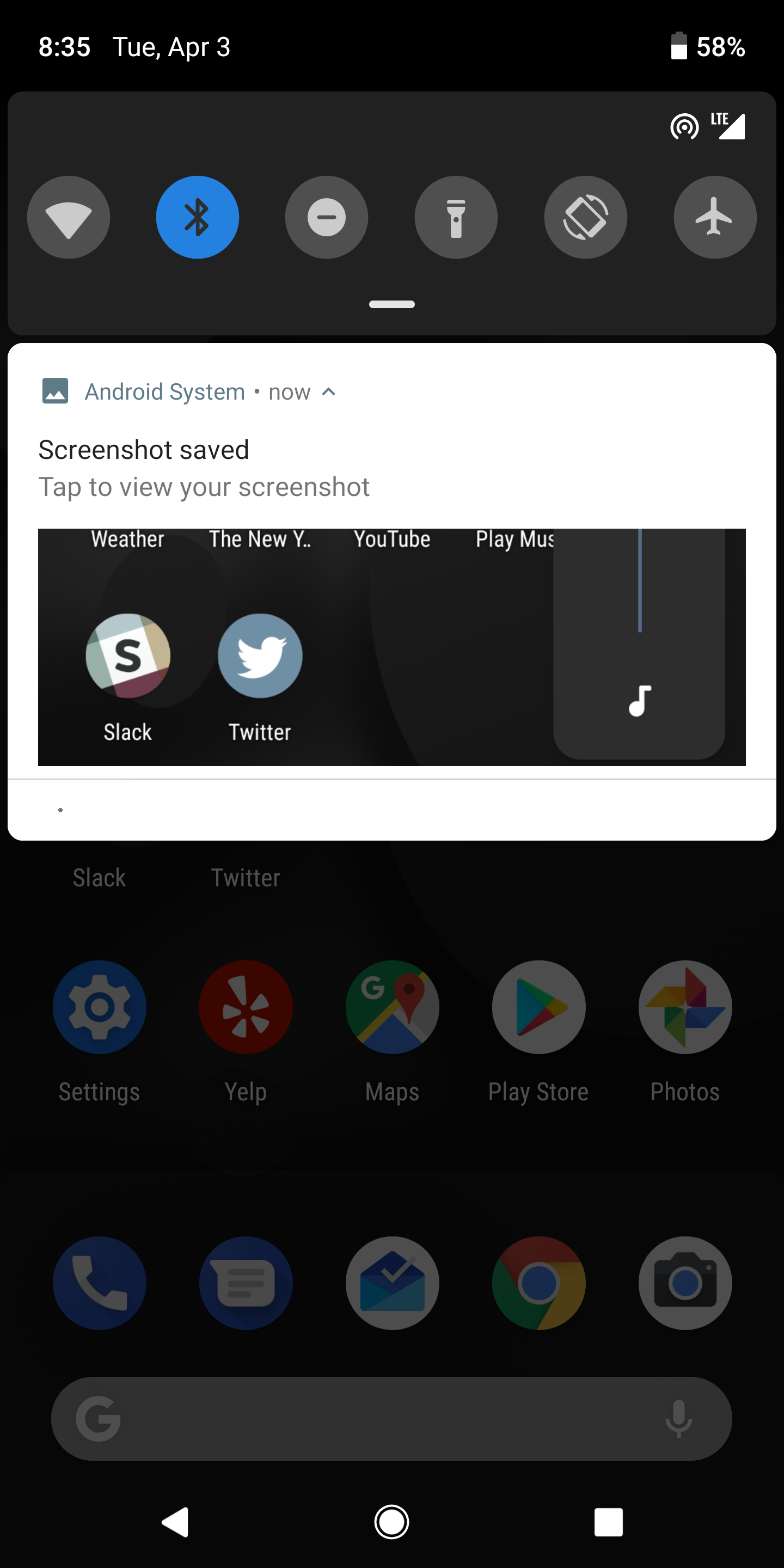A screenshot of an Android device home screen, showcasing various app icons and system notifications. At the top of the screen, the status bar displays indicators for Wi-Fi, Bluetooth, and other system statuses. The home screen is populated with several app icons including prominently displayed Slack and Twitter, which are highlighted by a notification stating "Android System - Screenshot saved. Tap to view your screenshot." Other visible app icons include Settings, Yelp, Maps, Play Store, and Photos, which appear slightly faded. Further down, there are icons for Telephone, Messages (depicted by a blue envelope with a white check mark), Chrome, and Camera. At the bottom, there is a long gray pill-shaped search bar available for text input.